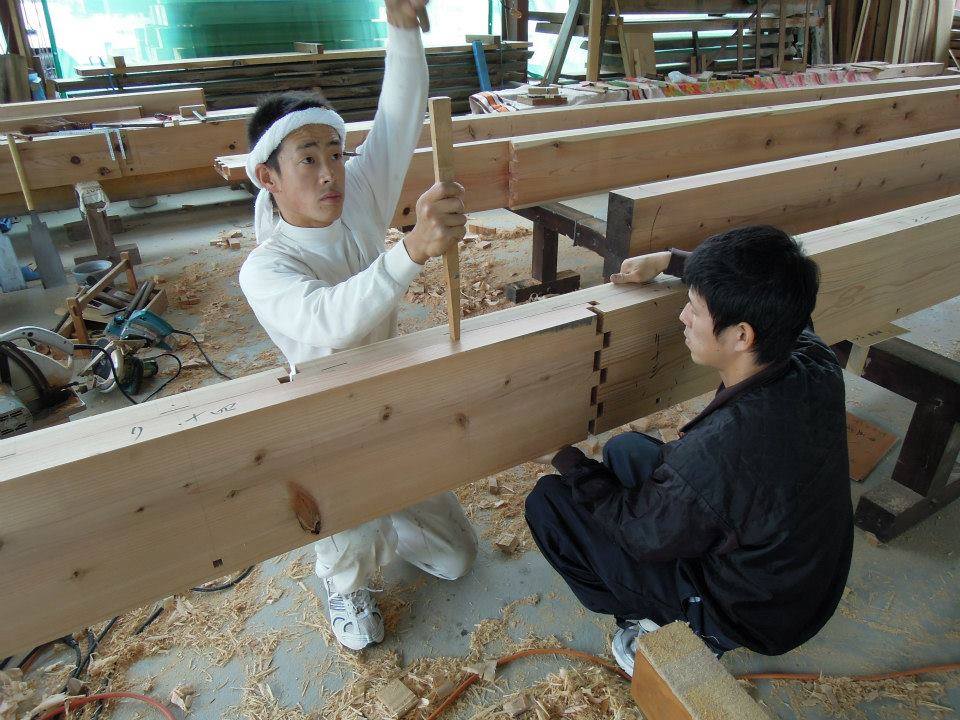In a well-lit woodshed bustling with activity, two Asian men are engrossed in a woodworking project during the daytime. The man on the left, dressed entirely in white with a band tied around his head, is actively hammering a pointy tool into a thick piece of wood, forming a cubic structure. Opposite him, the man dressed in all black, from his shirt and trousers to his hair, steadies the wooden piece on a table. Both men wear matching white sneakers. The floor is strewn with sawdust and wood chips, indicative of ongoing craftsmanship. The surroundings reveal a myriad of woodworking tools and equipment, including saws and saddle horses. Alongside various wooden structures and stacks of 2x4s, numerous long pieces of wood are being worked on or neatly stacked on racks and tables. In the midst of all this, two wolves lie on the ground on the left side of the image, their presence an intriguing addition to the industrious scene. The backdrop of the workshop, with its wooden materials and tools, frames the diligent focus of the two craftsmen.